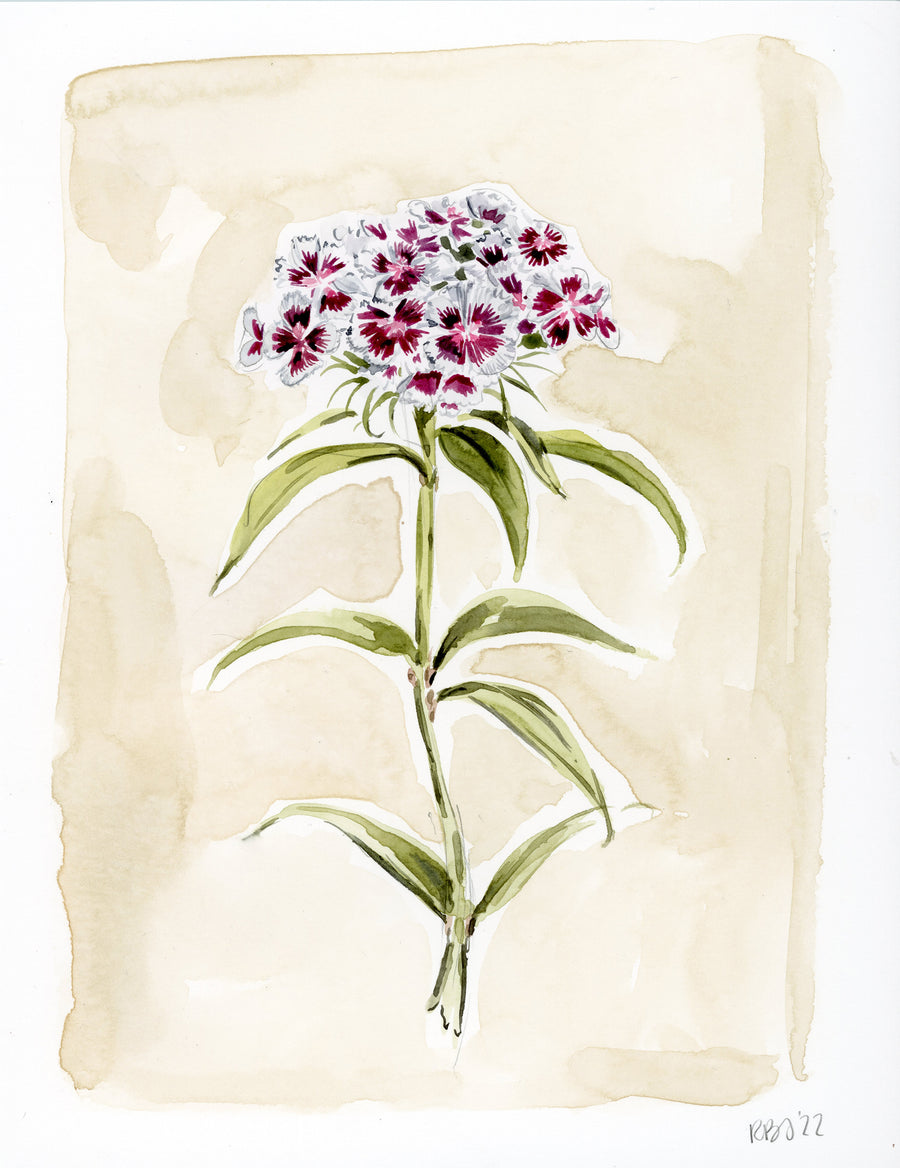This detailed watercolor painting depicts a single plant with a tall, olive-green stem, adorned with about 10 long, thin, pointed leaves, alternating on each side. At the crown of the stem, a lush collection of dianthus flowers blooms in varying shades of pinks, reds, and whites. The flowers exhibit burgundy centers that delicately fade to white towards the edges. The plant is set against a light beige background, giving it an antiquated, parchment-like appearance. The bottom corner of the painting is signed "RBS 22," adding a personal touch to this striking botanical artwork.